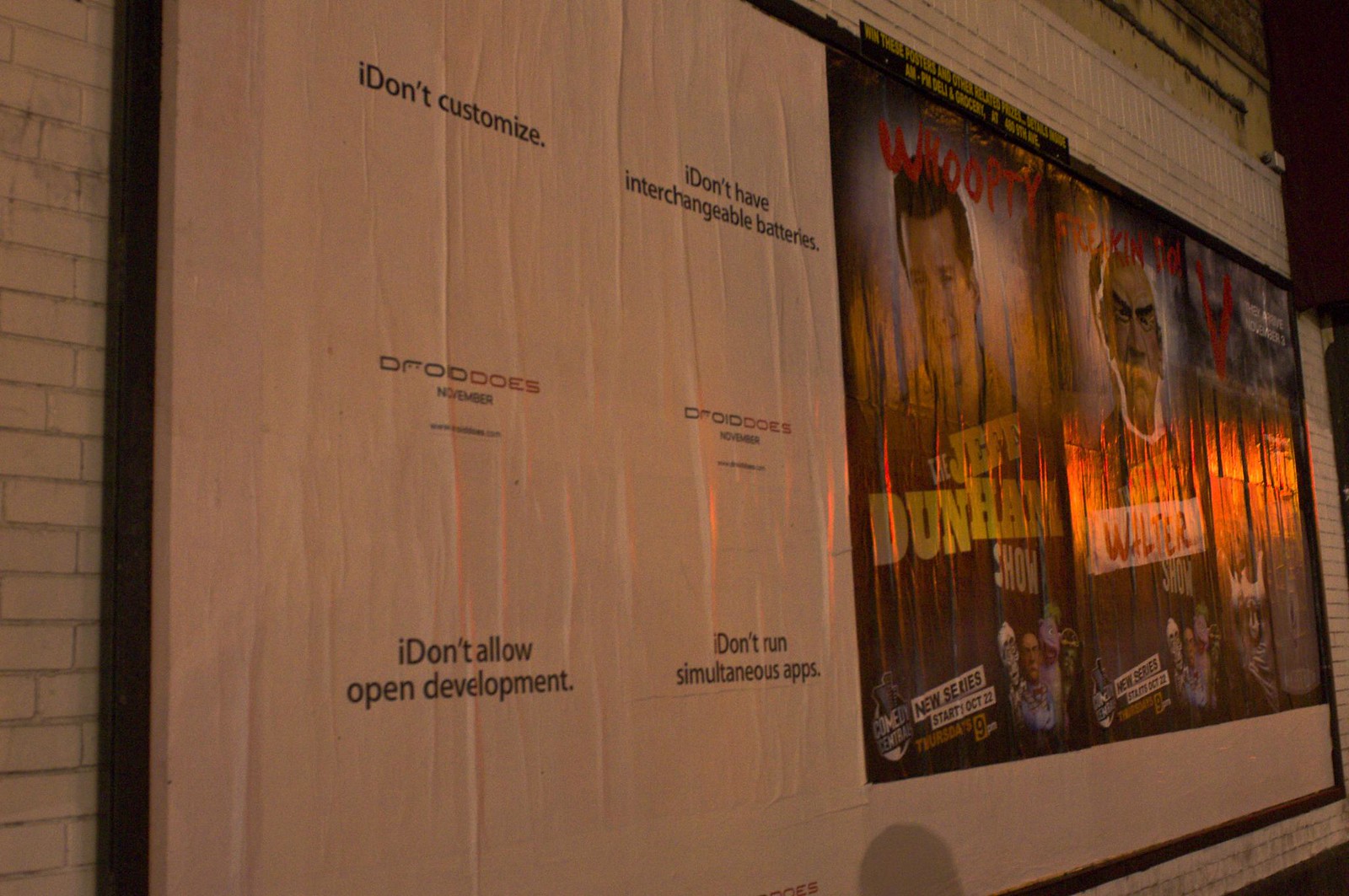The image showcases a series of advertisements mounted on a large, white brick wall outside, taken at an angle in low light, which adds a slight challenge to reading the content. On the left side, there are four wrinkled posters, each with black lettering on a white background, proclaiming messages like, "I don't customize," "I don't have interchangeable batteries," "I don't allow open development," and "I don't run simultaneous apps." Below each of these statements, there's the phrase "Droid does, November." To the right, three more advertisements are visible, including two promoting "The Jeff Dunham Show." One of these features a puppet named Walter, with red spray-painted lettering at the top saying, "whoopty frickin' do." At the bottom, the advertisement notes that a new series starts on October 22, airing Thursdays at 9 PM on Comedy Central. The combination of these details forms a comprehensive and detailed portrayal of the scene captured in the photo.